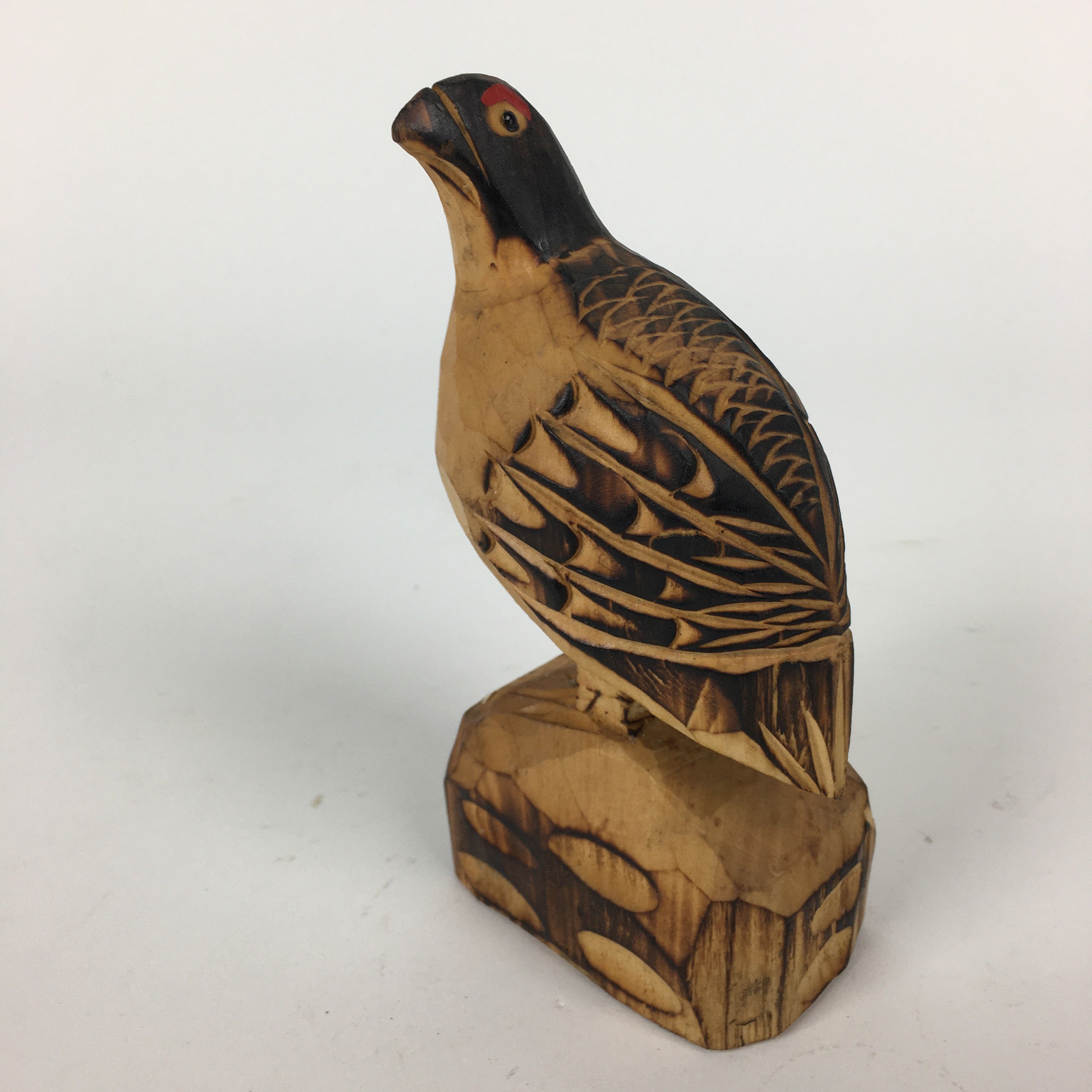The image showcases a beautifully crafted wooden statue of a bird, possibly a pigeon or a pheasant, perched on a sturdy, rectangular hardwood base. The base features elegant, darker brown swirled markings against a lighter brown backdrop, with dimensions approximately four inches by four inches and a thickness of one to two inches. The bird's head is black, adorned with a tan eye that has a black pupil and a distinctive red eyebrow. The bird is positioned to face the left side of the image, gazing upwards and slightly towards the camera, highlighting the left side of its head and a single eye. Its belly exhibits a pale, gold-tan wood, transitioning to darker brown with intricate feather markings down its back and wings, which include touches of gold. The entire statue rests on a plain white surface, under lighting that casts soft gray shadows, emphasizing the delicate and detailed workmanship of this exceptional piece.